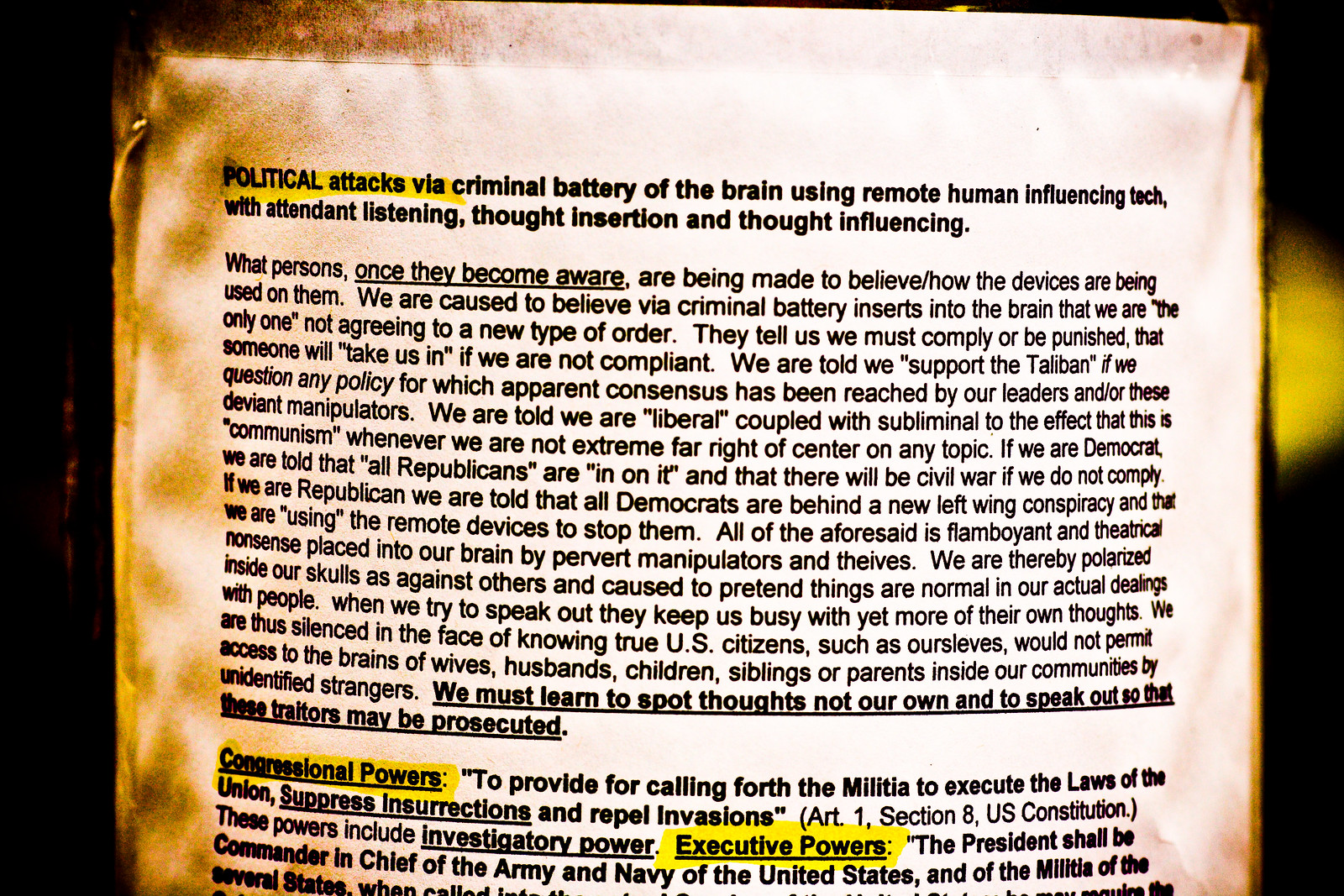The image depicts a piece of paper that appears to have been removed from a book or pamphlet, with noticeable burning or discoloration on the edges, particularly on the left, right, and top sides. The background of the image is black with some areas of yellow. The paper itself has distinct yellow and black stains in the top left corner and down the left side. 

The top of the page prominently features a heading in highlighted or outlined yellow letters that reads, "Political Attacks via Criminal Battery of the Brain using Remote Human Influencing Tech with Attendant Listening, Thought Insertion, and Thought Influencing." The rest of the text on the page is in black letters.

Beneath this heading is a detailed paragraph discussing the purported use of remote human influencing technology as a means of political control. It claims that individuals are subjected to thought insertion and are manipulated into believing they are isolated in their dissent against a so-called "new type of order." The narrative states that non-compliance leads to threats of punishment and that dissenters are accused of supporting the Taliban, being communist, or being part of left-wing or right-wing conspiracies, depending on their political alignment.

At the bottom of this paragraph, underlined in black, is a call to action: "We must learn to spot thoughts not our own and to speak out so that these traitors may be prosecuted."

Following this, a heading titled "Congressional Powers" appears, highlighted in yellow. The text underneath this heading is partially cut off at the bottom of the image, but it begins to discuss the constitutional powers granted to Congress, including the power to call forth the militia and execute the laws of the Union. There is also a mention of executive powers related to the President as the Commander-in-Chief of the Army and Navy.

The overall impression is of a politically charged document warning about alleged government or external manipulative tactics involving advanced technology to control individuals' thoughts and actions.